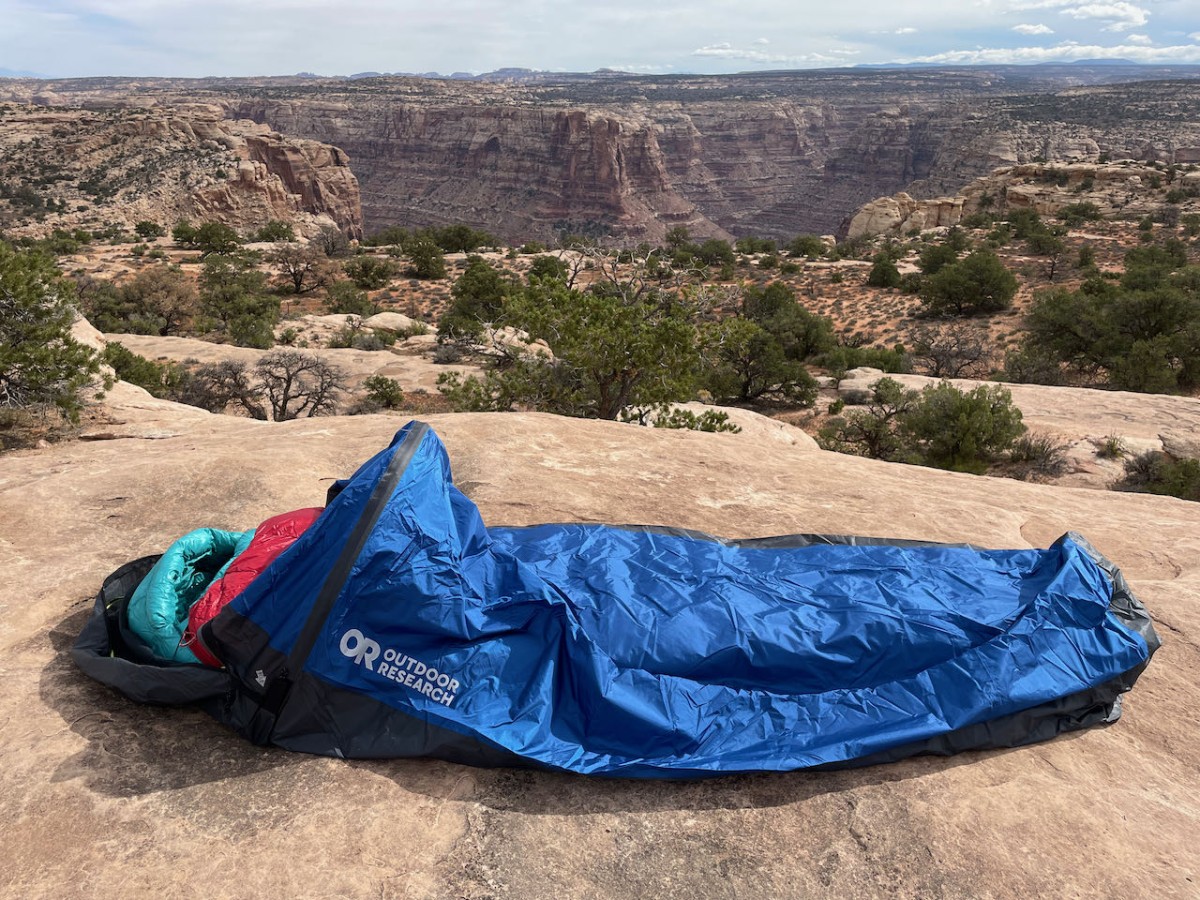A striking photograph captures a lone adventurer nestled in a turquoise sleeping bag with a red liner, all encased in a blue Outdoor Research bivy tent. The camper is perched atop a boulder, overlooking a vast, rugged valley that stretches into the distance. The valley features a washed-out rocky terrain interspersed with sparse green bushes. The landscape extends into a sweeping flat plain, with distant outlines of mountains or clouds creating a dramatic backdrop. Just a hint of the adventurer's hair peeks out from the top of the sleeping bag, which is oriented left to right across the boulder, emphasizing the scale and solitude of their breathtaking vantage point.